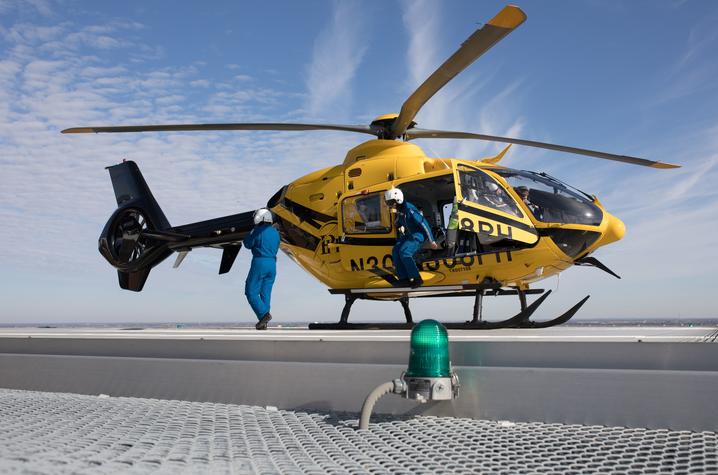The image captures a professional shot of a yellow and black helicopter with gray stationary blades, landed on a silver metal mesh platform which appears to be a designated helipad atop a building. In the foreground, there is an unlit green bulb light on the platform. The helicopter bears the text "N308 RH" on its door, although it is somewhat difficult to discern. The setting includes a background of fluffy white clouds against a yellowish hue, suggesting high altitude. Onboard, a pilot with a white helmet is visible through the windshield. Two individuals in blue jumpsuits and white helmets are disembarking; one is exiting via the open door while the other heads toward the helicopter's tail. The upper right of the background features a deep blue sky that transitions to more cloudiness towards the left and downward, adding to the high-altitude impression.